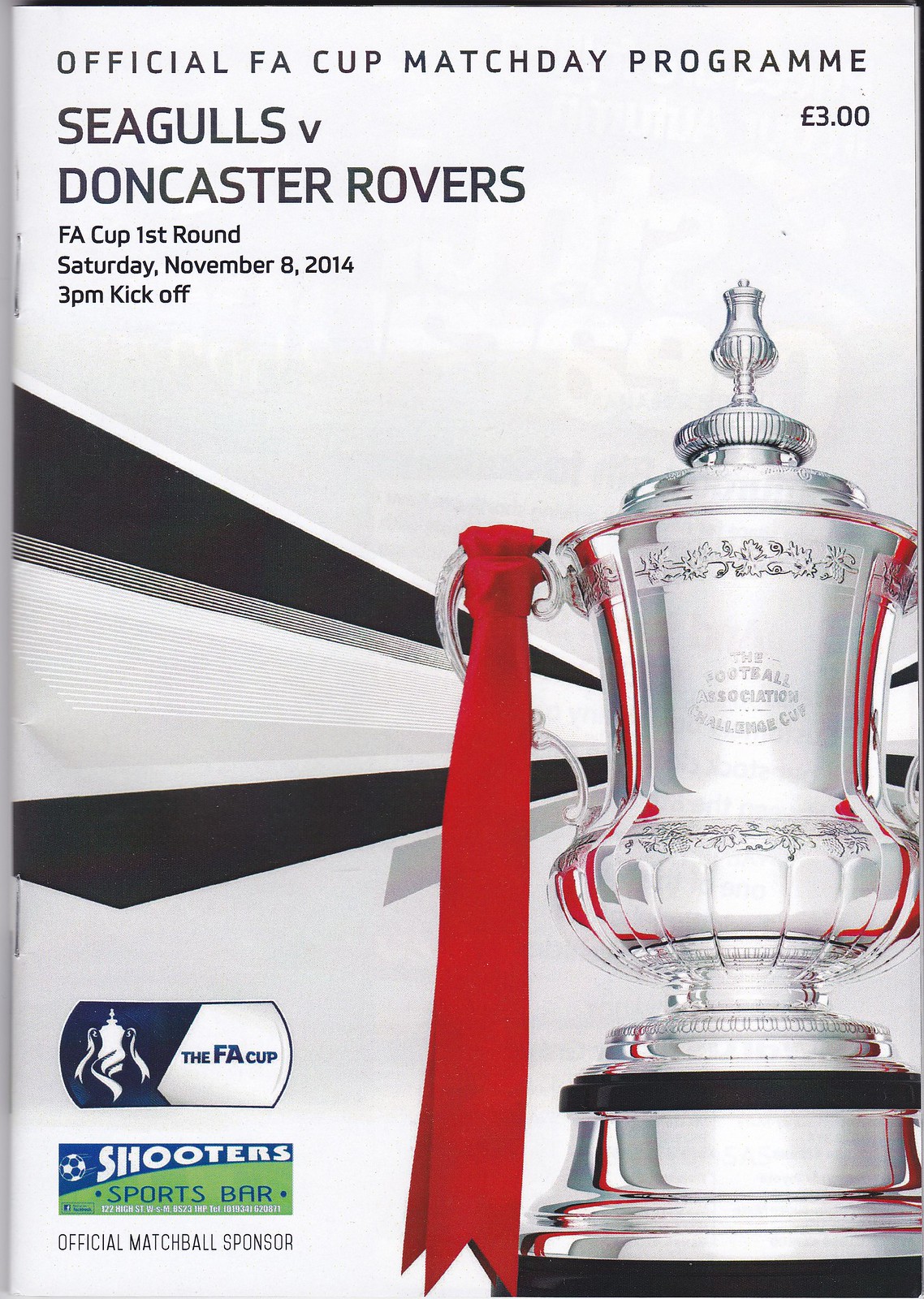The image is an advertisement for a sports event featuring the Official FA Cup Matchday Program. The text at the top announces the FA Cup first round match between Seagulls and Doncaster Rovers, scheduled for Saturday, November 8, 2014, with a 3 p.m. kickoff. The program costs 3 Euros. Dominating the right side of the image is a silver trophy adorned with a red ribbon on one handle. Below the trophy, the FA Cup logo is visible. Additionally, the advertisement promotes Shooters Sports Bar within a blue and green rectangle and mentions the world's official matchball sponsor in black text at the bottom.